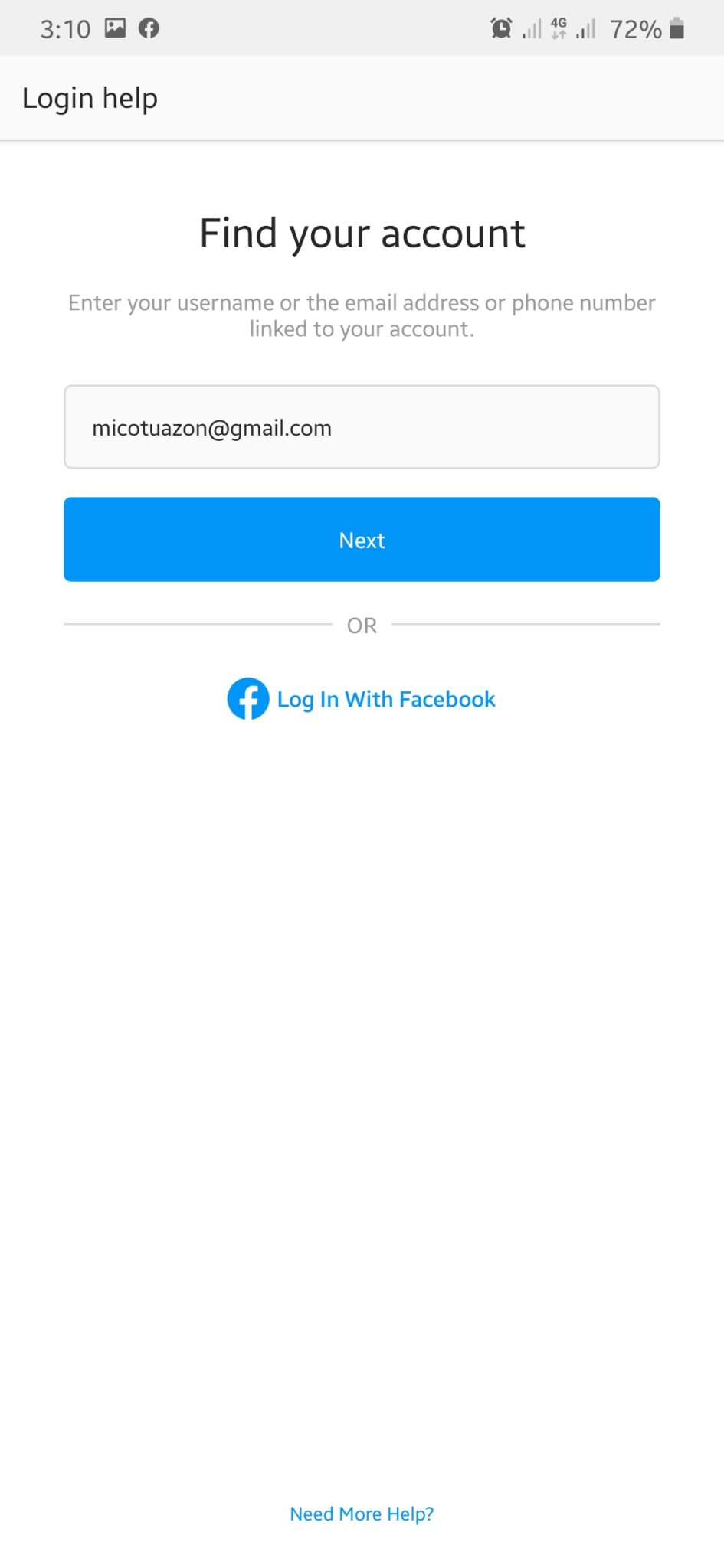The image depicts a smartphone screen displaying a user's attempt to log into their Facebook account. At the top of the screen, the standard status bar shows the time as 3:10 PM. The icons present include a photos icon, a Facebook icon, and an alarm icon. The phone shows a weak signal strength with one bar, but it also displays "4G" and two bars next to each other, indicating some level of connectivity. The battery icon indicates a charge level of 72%.

At the upper section of the screen, there's text that reads "Log In Help." Below that, in the center of the screen, on a white background with black text, it says "Find Your Account." Underneath this, in smaller, grey text, it instructs the user to "Enter your username or the email address or phone number linked to your account."

A text input field has been filled with the email address "micotuazon@gmail.com." Below this input box, there is a prominent "Next" button followed by the word "or" with a horizontal line. Another option provided is to "Log In with Facebook," accompanied by the Facebook icon. At the very bottom of the screen, a clickable blue text reads "Need more help," offering additional assistance options.

This detailed layout ensures the user has multiple options and clear instructions for logging into their Facebook account or seeking further help if needed.